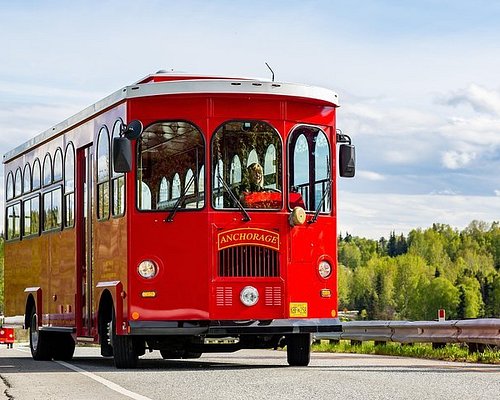This landscape-oriented photograph captures a vintage red bus styled to resemble a classic trolley, complete with wheels for road travel rather than tracks. The bus, emblazoned with "Anchorage" in golden letters at the front, features rounded windows all around, enhancing its charming old-fashioned appearance. White trim adorns the top edge, adding a touch of elegance. This bus, possibly used for tours, appears to be in well-maintained condition as it traverses a gray asphalt road. In the driver's seat, a woman with blonde hair is visible, navigating a turn as evidenced by the angled front wheels. The surroundings reveal a sunny day with blue skies and light, fluffy clouds. To the left, lush green trees and a highway guardrail are visible, contributing to the picturesque setting, likely somewhere in Alaska.